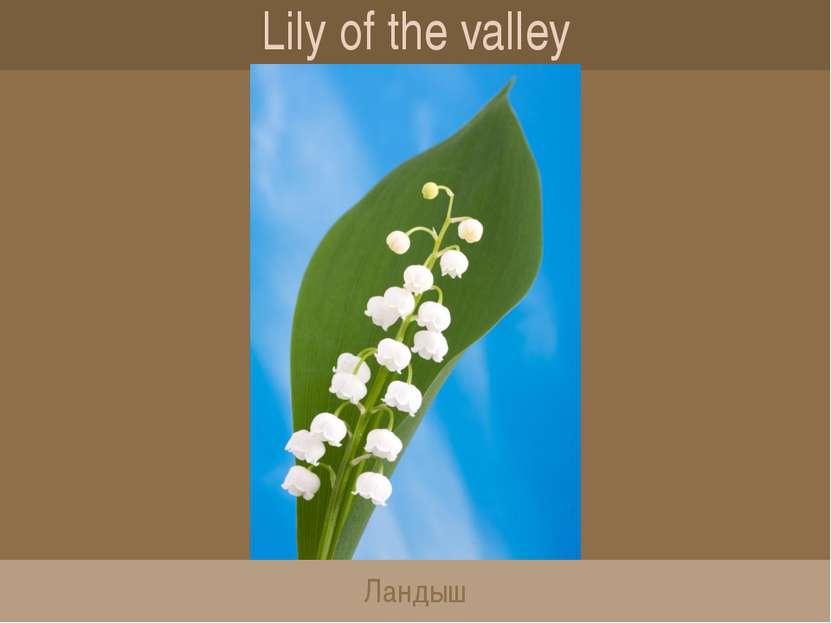The image features a meticulously detailed sketch with a beautifully arranged layout. It consists of a solid brown background framed by narrow horizontal strips. At the very top, a darker brown strip contains the centered phrase "Lily of the Valley" in light beige lettering. Below this, in the middle section, is an elongated rectangle depicting a bright blue sky with subtle, faint white clouds, serving as a serene backdrop.

In the foreground of this central rectangle, a verdant green stem features an elegant array of white, bell-shaped Lily of the Valley flowers. The flowers have a delicate, drooping posture, pointing towards the ground, with the blossoms near the bottom of the stem appearing more open and in full bloom, while those higher up remain more tightly clustered. A single, elongated green leaf adds to the natural beauty, stretching out beneath the flowers.

At the bottom of the image is another narrow horizontal strip in a taupe color. Centered within this strip are enigmatic symbols, resembling "N-A-H," an odd symbol, "B-L," and a prominent "W," though their meaning remains unclear. Overall, the sketch conveys a sophisticated and peaceful scene, highlighted by the graceful Lily of the Valley flowers.